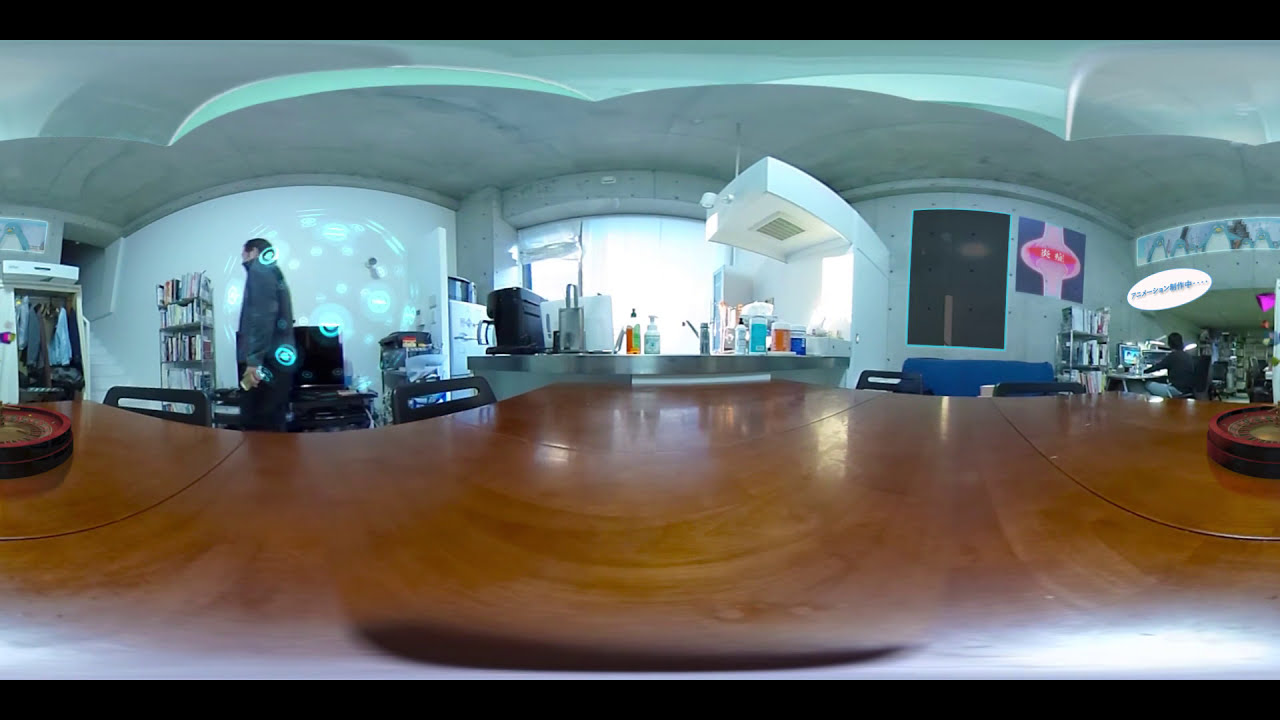This blurry, fisheye-lens photograph appears to be taken indoors, possibly in a restaurant, office, or shop setting. The foreground contains a large, finished woodgrain table with reflections on its surface. To the left edge, there's a Caucasian man in dark attire possibly walking by, framed against a bookcase. The central background reveals a window flooding the space with daylight, suggesting it is the middle of the day. The white walls feature signs with Asian characters in purple and pink, and a digital screen is visible on the right side. There are various objects on a counter including lotions or soap, implying a makeup counter or cafeteria setup. Someone is seen seated at a desk or table, focused on a computer. The ceiling appears to be cement, and there are no artificial lights on, with all luminosity coming from outside. The overall scene presents a cluttered but detailed environment bathed in natural light.